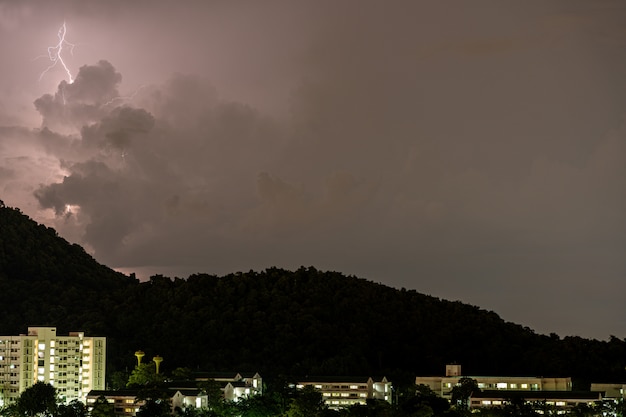This nighttime photograph captures a dramatic thunderstorm scene over a cityscape. Dominating the left side of the image, a powerful bolt of lightning strikes from the purple-tinged clouds, illuminating the sky in shades of light purple and gray. The lightning's branches radiate across the sky, creating an electrifying spectacle. Below, the foreground features a collection of white buildings, most notably a tall structure with approximately seven to ten stories on the left. Surrounding this high-rise are several smaller buildings, ranging from three to four stories, all of which have some illuminated windows casting a warm, yellow light. Behind these buildings lies a hill or mountain range, largely shrouded in darkness and appearing almost black, which ascends higher towards the left and gradually lowers to the right. Tall palm trees are interspersed among the buildings, adding to the nocturnal landscape. The overall scene is rendered with striking contrast due to the stormy weather and is likely captured using time-lapse photography to perfectly freeze the moment of the lightning strike.